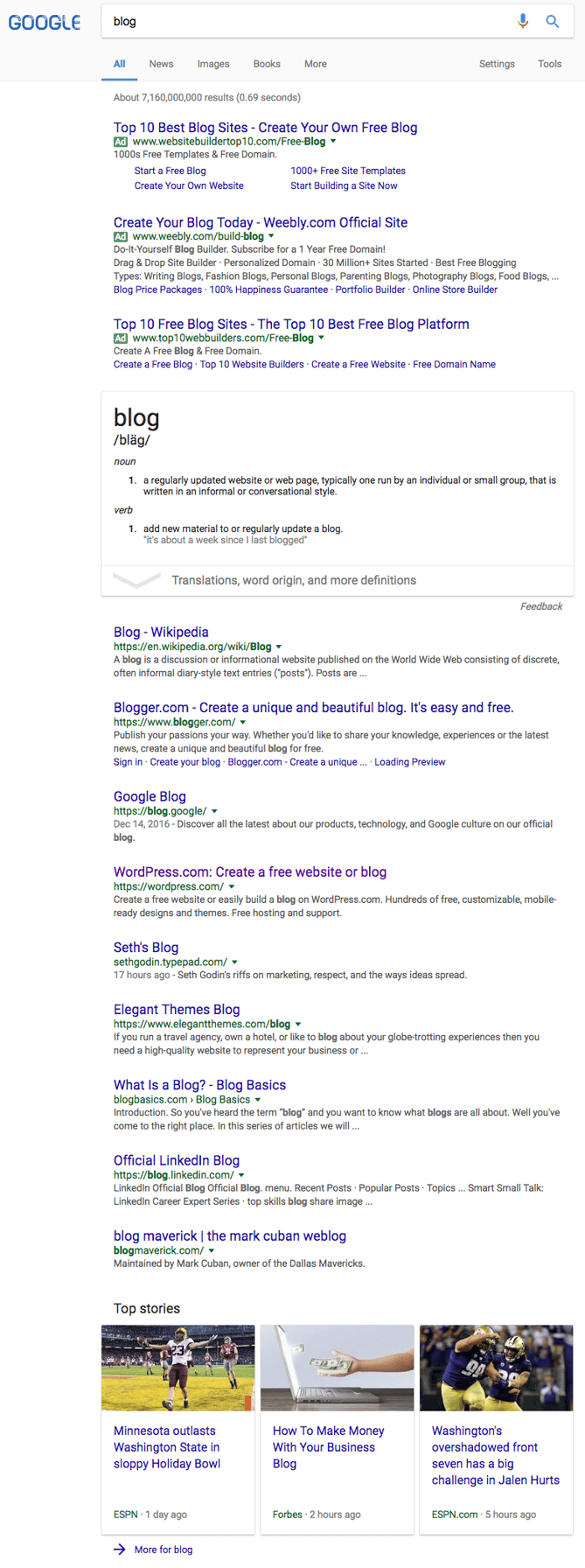Screenshot of Google Search Results for "Blog"

The image is a screenshot of a Google search page. At the top left corner, the Google logo is distinctly different, appearing in an all-blue color scheme, which is larger and wider than usual, possibly indicating a special event or theme on that day. The search query entered in the search bar is the single word "blog."

The search results begin with three advertisements. The first ad is titled "Top Ten Best Blog Sites - Create Your Own Free Blog," the second one reads "Create Your Blog Today - Weebly.com Official Site," and the third ad states "Top Ten Free Blog Sites - Top Ten Best Free Blog Platform."

Following the ads, the first organic search result presents the definition of the word "blog," defined as "a regularly updated website or webpage, typically run by an individual or small group that is written in an informal or conversational style." Additional search results include links to a Wikipedia article on blogs, blogger.com, Google's blog, and wordpress.com, the latter of which is shown in purple, indicating that it has been previously visited by the user.